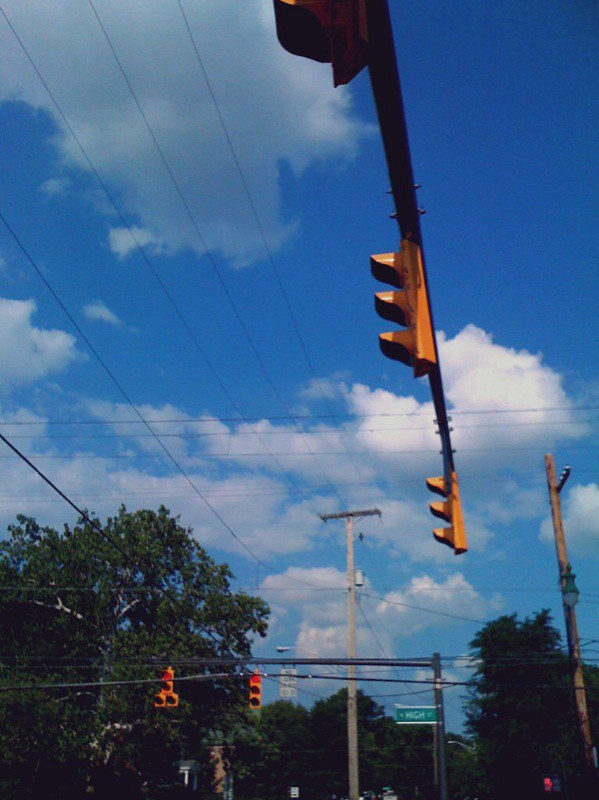The image features a vibrant urban scene taken from the perspective of someone standing beneath traffic lights at an intersection. The traffic signals, visible in both directions, indicate that the lights directly across the street are red, while those parallel to the viewer's position show green. This suggests a multi-lane road, given the several signal lights present.

Overhead, power poles extend across the scene, and a street sign on the opposite side of the intersection identifies the perpendicular road as High Street. The sky is a brilliant blue adorned with fluffy white clouds, reflecting a bright and sunny day. Verdant green trees, likely deciduous, line the street, indicating that the photo was captured during spring or summer.

Shadows cast from the poles appear to stretch across the road, suggesting the sun is situated behind the photographer. This detailed interplay of elements creates a scene vivid with life and natural beauty, captured on a perfect day.